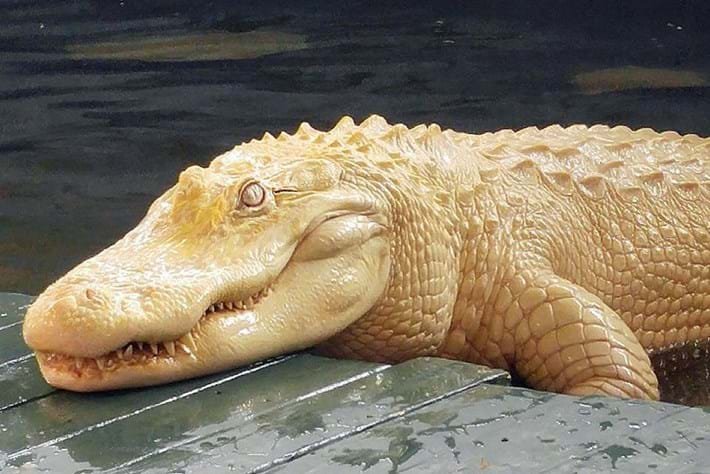This is a horizontally aligned rectangular photograph of an albino crocodile with a light beige or whitish-yellow body and some yellow tint on the top of its head. The crocodile's eye blends with the body color, making it appear closed or shaded, and its teeth are visibly overlapping its closed mouth. The crocodile's head is resting on gray, weathered wooden planks of what appears to be a pier or bridge, with wet marks indicating it just emerged from the water. The top of the picture features a mix of black, gray, and brown shades, and the scene suggests an outdoor setting, possibly an enclosure. The majority of its body remains in the shallow, gray or blue water in the background, creating a natural yet striking contrast with the dry wooden surface.